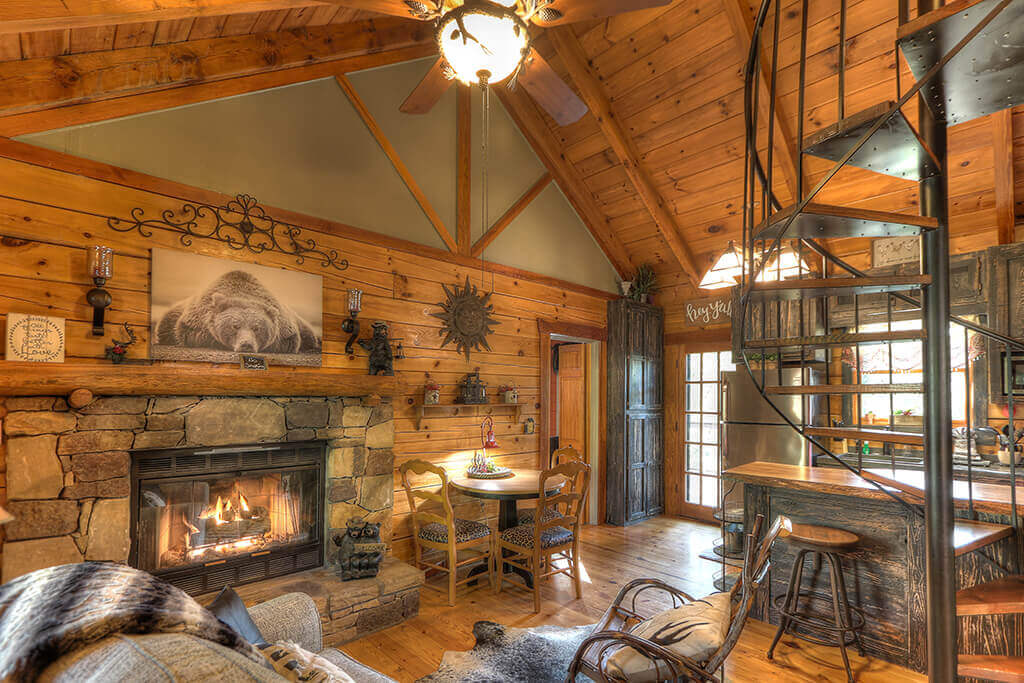This detailed interior photograph captures the cozy ambiance of a rustic log cabin, entirely clad in medium-stained wood. Dominating the center of the room is a stone fireplace with a burning fire, which is encased in black trim and adorned above with a striking black and white picture of a bear, flanked by side lights. Nearby, a wooden rocking chair sits atop a bear fur rug, enhancing the rustic decor that permeates every corner of the cabin. The room also features a round iron staircase with wooden steps leading to an upper level, positioned near a kitchen area equipped with a stainless steel refrigerator. On one side, a wooden bar is paired with a matching stool, perfect for casual seating. Overhead, a rustic ceiling fan accentuates the room's charm, and a glow light hangs from the ceiling, bathing the space in warm light. Additional furniture, including a couch and a small round table with chairs, is arranged to create a welcoming and comfortable atmosphere, while the sunlight streaming in from outside adds to the room's inviting feel.